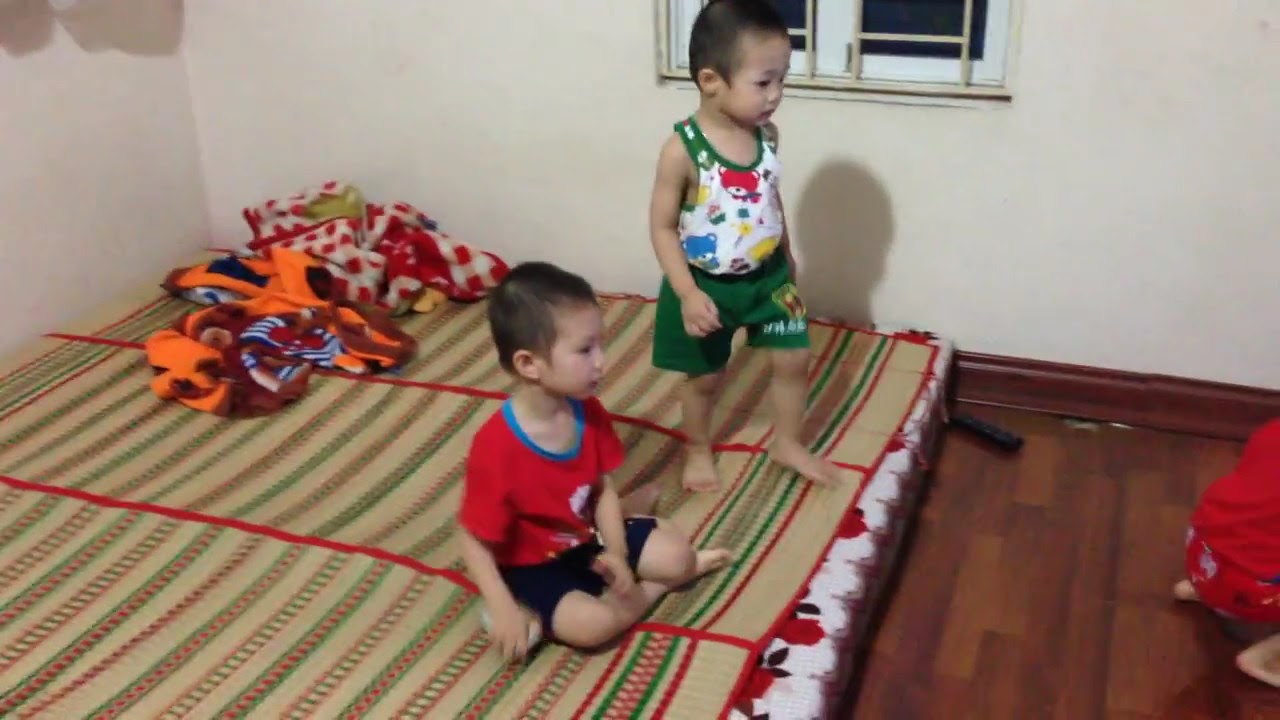This indoor image depicts three young children, likely toddlers, centered around a mattress placed on a dark wooden floor. The primary focus is on two boys on the mattress; the one seated is dressed in a red t-shirt with a blue collar, dark shorts, and has short black hair. Next to him, slightly behind and standing, is another boy in a white sleeveless tank top with green trim and bear designs in blue and red, paired with green shorts. Both boys are gazing towards a third child, who is mostly cropped out of the image, crouched on the floor to the right, wearing a matching red shirt and shorts. The setting includes a cluttered corner with blankets in various colors—green, brown, red, and white—and a cream-colored wall with some brown paint visible. A pair of windows can be seen behind the standing boy, and a black remote control lies beside the mattress. The overall scene is busy and colorful, reflective of a playful, child-centric environment.